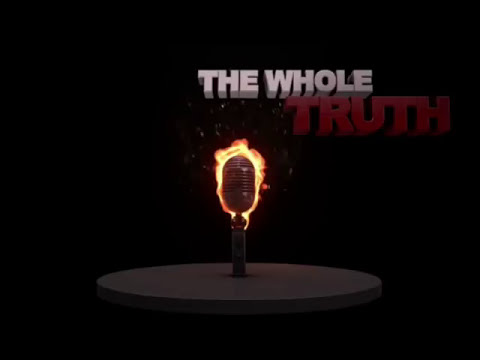This graphic design image, possibly created using software such as Adobe Photoshop, depicts a dramatic and dark scene primarily featuring a single, old-school silver microphone on fire with intense orange and yellow flames and embers rising up. The microphone is centrally positioned on a circular, stone or concrete-like gray platform, which occupies the bottom center of the composition. The background of the image is predominantly black, adding to the intensity of the fiery microphone as the focal point. In the top right corner, bold text reads "The Whole Truth" with "The Whole" in white and "Truth" in red, both featuring a 3D effect that stands out against the dark background. This image likely represents an advertisement for a talk show, emphasizing fiery, unfiltered honesty.